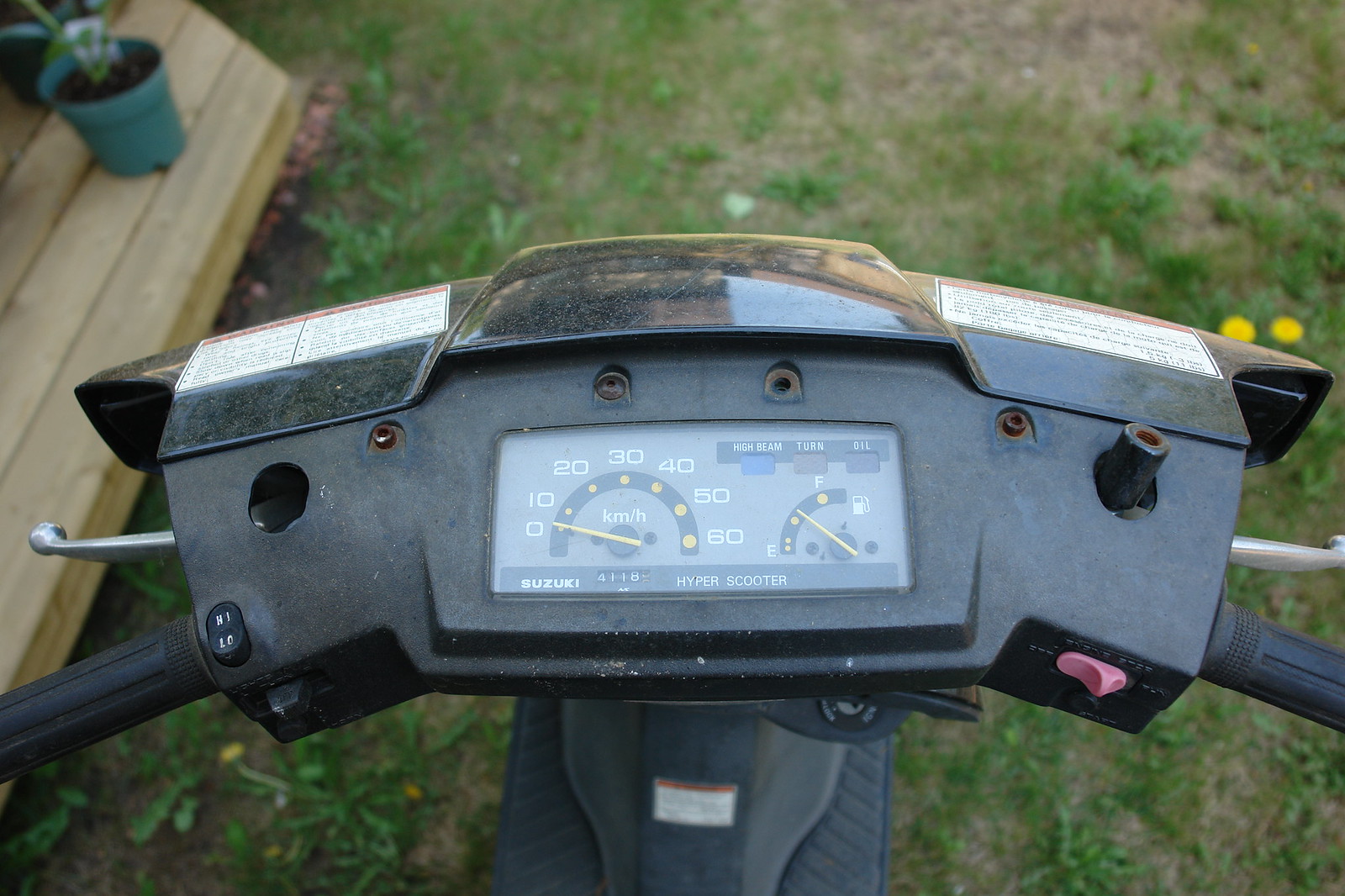A detailed image description:

The photo captures the central section of a motorized scooter or motorcycle, prominently displaying the speedometer and fuel gauge. The speedometer, with numbers ranging from 0 to 60, is the focal point, indicating a bit over half a tank of gas remaining, with markers at 'E' (Empty) and 'F' (Full). Below and to the right of the speedometer, there's a red on/off button, indicating the vehicle is powered. Surrounding the speedometer and fuel gauge is a black plastic housing, slightly dusty as if the vehicle has been stored in a garage for some time.

In the background, there's a patch of green grass with three visible yellow dandelions. To the right side of the image, a wooden patio is partially visible, along with a green plant in a pot. The black section where the rider would place their feet is visible in the lower part of the image, along with the black support for the handlebars. The scooter also has a protective plastic cover over the speedometer and fuel gauge to prevent bugs and debris from hitting them while riding.